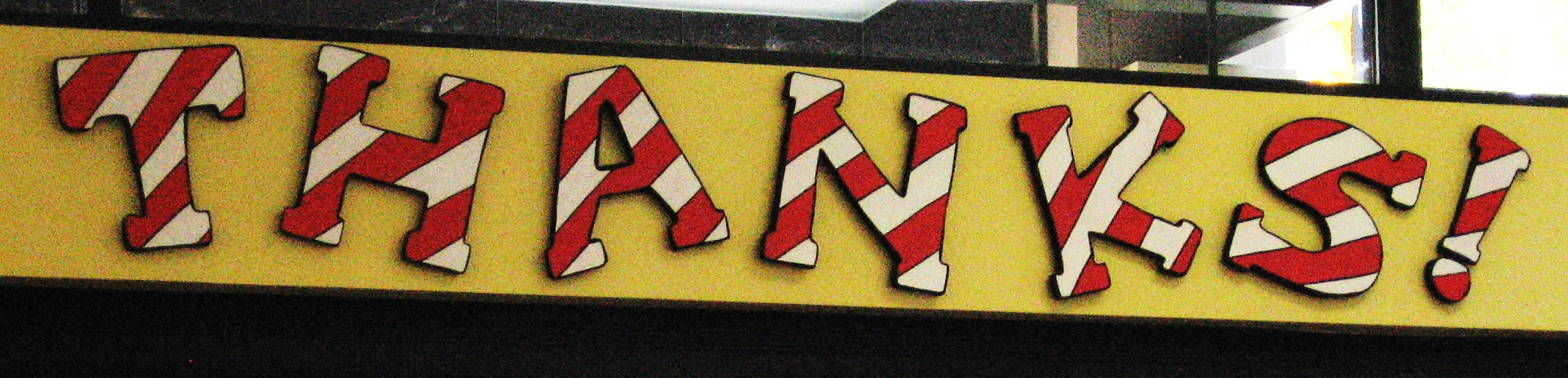This is a color photograph featuring a yellow, oblong-shaped sign with the word "THANKS!" written in capital letters across the center. Each letter of the word, as well as the exclamation mark, is decorated with diagonal red and white stripes, giving them a candy cane-like appearance. The text is slightly tilted but reads from left to right. The sign itself occupies most of the photo, standing out against a black background that frames its sides. At the top left corner of the image, there is a small portion of what appears to be a building with a window, showcasing a brown interior and a black exterior.